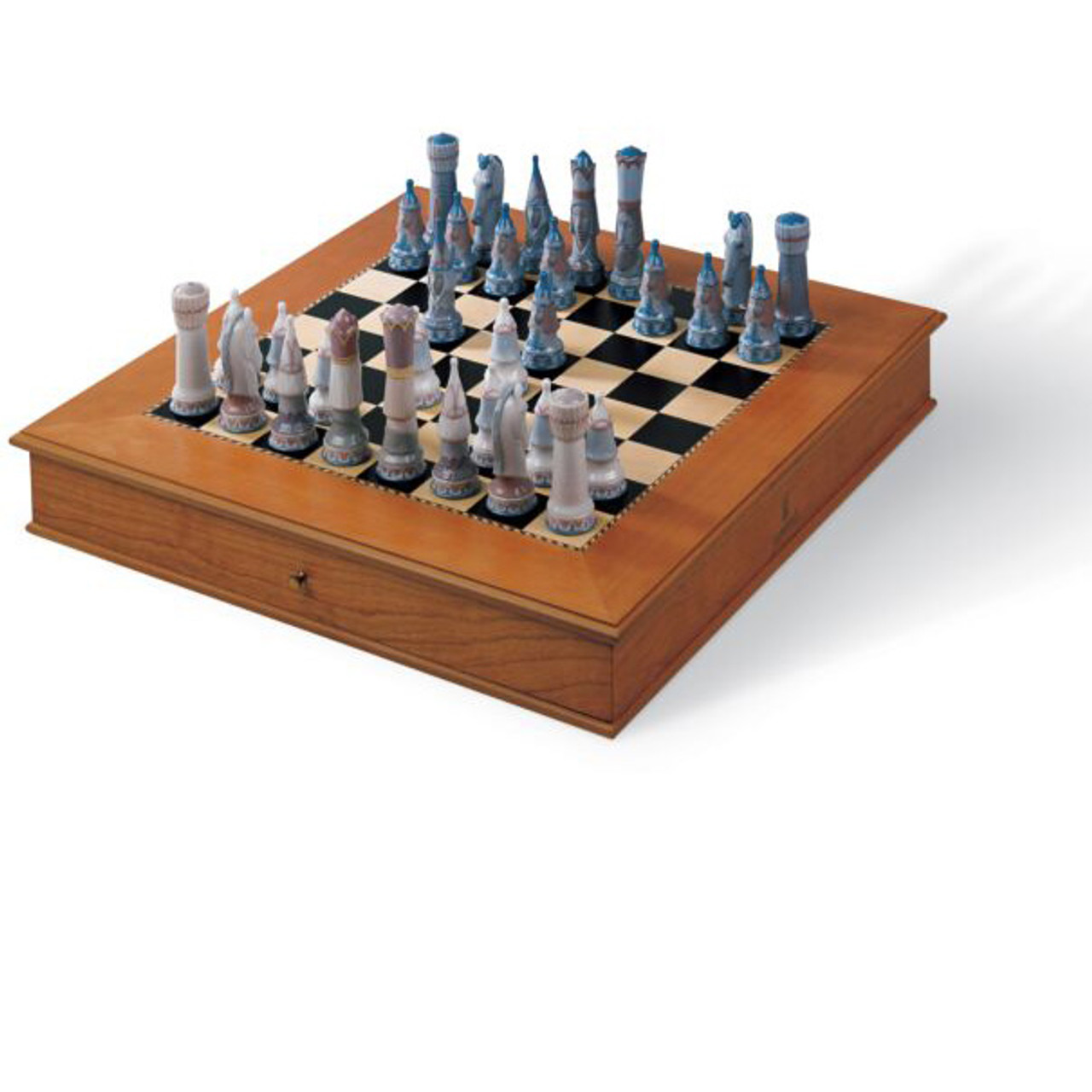This photo showcases a sophisticated and modern chess set that combines elegance with functionality. The chessboard is a black and white checkered pattern, crafted as part of a wooden, dresser drawer-like unit, complete with a knob, suggesting it can be opened to store the pieces inside. The pieces themselves appear expensive and potentially fragile, resembling carved stone or marble. 

Each side's pieces are striated with distinctive colors: the light side features shades of light gray, tan, and perhaps light lavender or brown, while the dark side comprises varying hues of gray, blue, darker mauve, or rust, with marbling details. The game is set up at the opening stage, with the two middle pawns on both sides moved forward one space. Overall, the raised square board and strikingly colored, ceramic-like pieces rest against a plain white background, adding to the clean and luxurious appearance of the set.